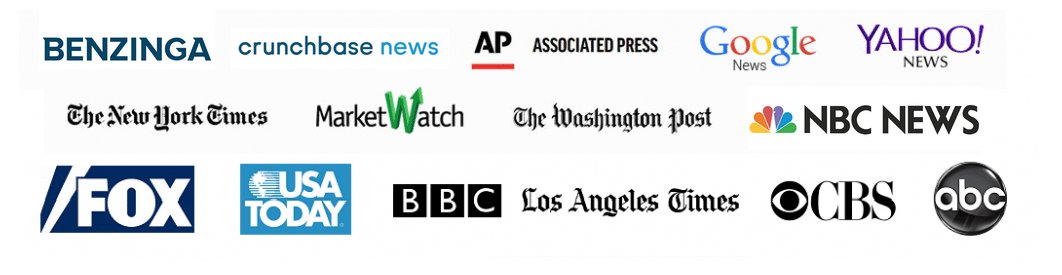The image is a collage of various news site logos on a clean, white background, organized neatly in rows. 

**Top Row (left to right):**
1. **Benzinga** - The logo appears prominently on the top left.
2. **CrunchBase News** - Next to Benzinga.
3. **AP** - Displayed in black with a red underline, followed by the words **Associated Press**.
4. **Google News** - Positioned right after the Associated Press logo.
5. **Yahoo News** - Marked in purple, finishing the top row.

**Middle Row (left to right):**
1. **The New York Times** - Starting the second row.
2. **Market Watch** - Notable for the green 'W' in the logo.
3. **The New York Post** - Located next to Market Watch.
4. **NBC News** - Identifiable by an adjacent image of the iconic NBC peacock with feathers in yellow, orange, red, purple, blue, and green.

**Bottom Row (left to right):**
1. **Fox** - Shown within a blue rectangle.
2. **USA Today** - Also in a blue rectangle to the right of Fox.
3. **BBC** - Presented within three black boxes.
4. **Los Angeles Times** - Following the BBC logo.
5. **CBS** - Accompanied by a circular eye-like symbol to the left.
6. **ABC** - Concluding with a distinct black circle displaying 'ABC'.

This detailed arrangement highlights a variety of major news outlets, offering a comprehensive visual representation of different media sources.